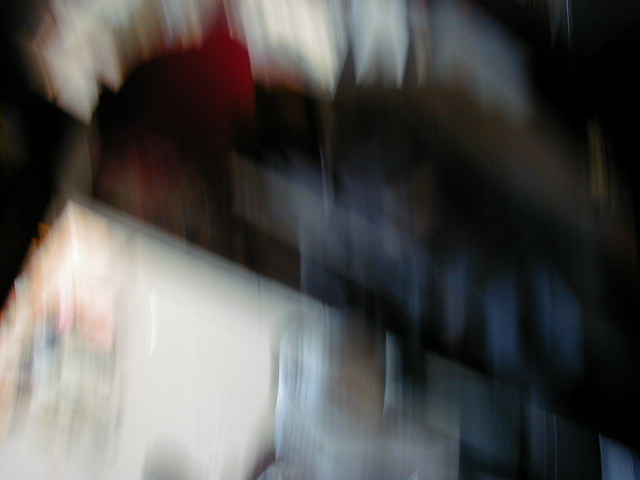The image, though extremely blurry and captured in motion, reveals a cozy indoor scene. At the center of focus is a dog, likely a husky mix, sitting attentively on the right side of the frame. The dog has a striking black and white coat, with erect ears that suggest he is intrigued by something his owner is saying. Despite the motion blur, the dog's eyes seem to be looking directly at the camera, capturing a moment of engaged curiosity.

In the background, indistinct shapes and colors suggest a domestic setting, perhaps inside a room of the house. A red streak, possibly from a toy, ascends upwards near the dog, adding a sense of dynamic movement to the scene. The lower half of the image is predominantly white, potentially indicating a piece of furniture like a table. Similarly, there is more white interspersed with shadows and darker areas in the background, which contribute to the ambient, somewhat enigmatic atmosphere of the snapshot.